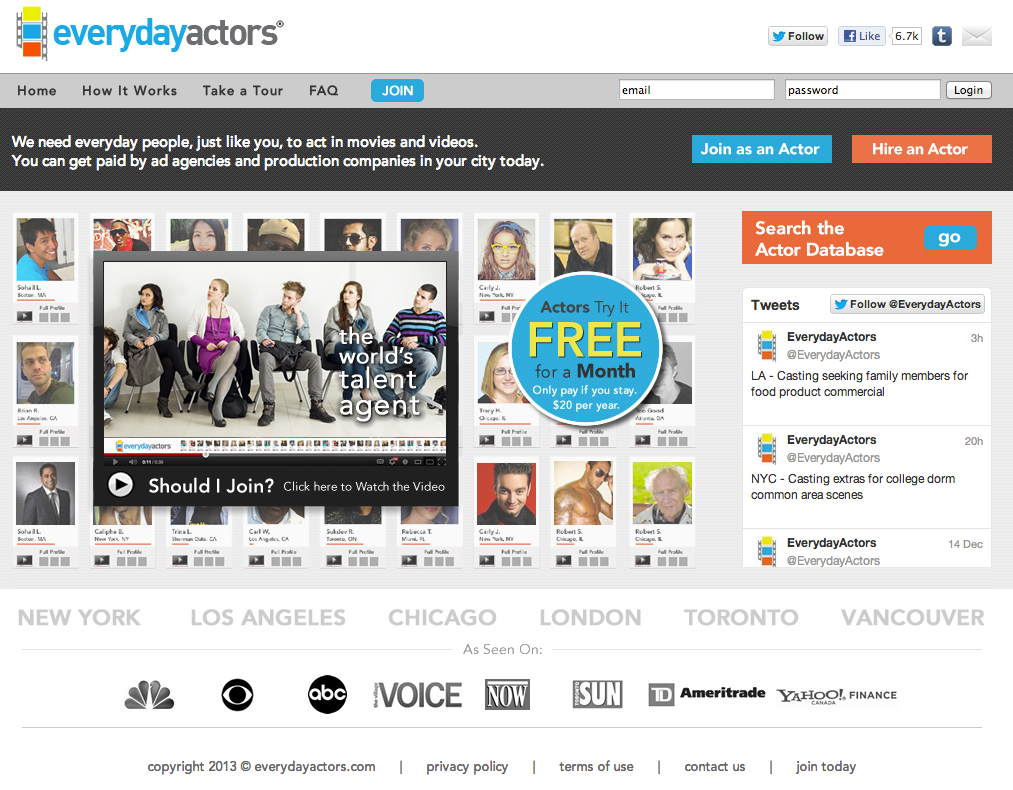This image is a screenshot from an online platform tailored for actors looking to sign up and get noticed by agents or casting directors for movies, television shows, and plays. 

At the top-left corner of the webpage, there's a colorful icon resembling a strip of celluloid film from old-school movie cameras, with black sprocket holes on the side. The film strip features yellow, blue, and orange squares where the film footage would be. To the right of this icon, in blue, it reads "Every Day" and to the right of that, in black, it says "Actors." 

In the top-right corner, a number of social media icons are visible, including Facebook and TikTok.

Directly beneath this header, a gray navigation bar stretches across the page with menu options listed from left to right: Home, How It Works, Take a Tour, and Join. To the far right of this bar, there are text fields for email and password entry alongside a gray login button.

On the main banner, there are two prominent call-to-action buttons: a blue button with white text that says "Join as an Actor" and an orange button with white text that reads "Hire an Actor."

The left-hand side of the page features a grid of small, identifiable photos of aspiring actors, each displaying their first name, last initial, photograph, and location. Overlaid on this grid is a pop-up box showing an image of five individuals seated as if at a casting call, with the text "The World's Talent Agent" alongside an invitation to watch a video titled "Should I Join? Click here to watch the video."

On the right-hand side of the page, there's a blue circle containing the offer: "Actors try it free for a month, only pay if you stay, $20 per year." Directly below this offer is an orange banner with a search button labeled "Search the Actor Database" and a blue "Go" button. Scrolling further down reveals a list of recent tweets from the Everyday Actors website.

At the bottom of the page, the cities New York, Los Angeles, Chicago, London, Toronto, and Vancouver are listed, followed by a line-up of logos from reputable organizations including NBC, CBS, ABC, Village Voice, NOW, Sun, Ameritrade, and Yahoo Finance.

The overall layout is designed to facilitate interaction and provide easy access to both aspiring actors and industry professionals.